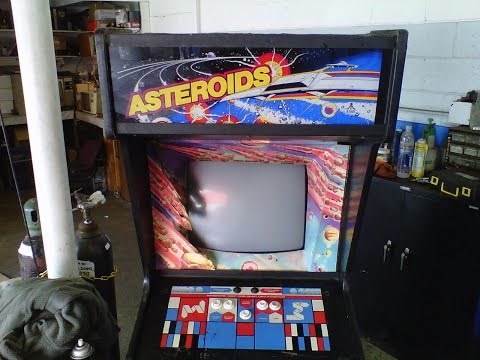The image captures a vintage Asteroids arcade game prominently displayed in someone's garage. The arcade machine itself is housed in an old-school black casing with a tube TV screen in the middle, currently turned off and appearing gray. The screen is surrounded by a colorful frame featuring a spaceship and an outer space theme, with "Asteroids" displayed in traditional yellow letters at the top. The control panel at the bottom features five white buttons set against a background of red, blue, and black squares.

To the left of the arcade machine, a tall white pole extends from the cement floor to the ceiling. The background reveals a white brick wall with clusters of wooden shelves in the left corner, cluttered with various items typical of a garage setting. On the right side of the photo, there are several black cabinets with silver handles, which likely serve as storage for tools or other equipment. Additional details in the background suggest a toolbox or tool chest, neatly stacked boxes, and some tanks, indicative of a space utilized for trade or workshop activities. The overall scene combines elements of nostalgia and practicality, blending a piece of gaming history with everyday garage organization.